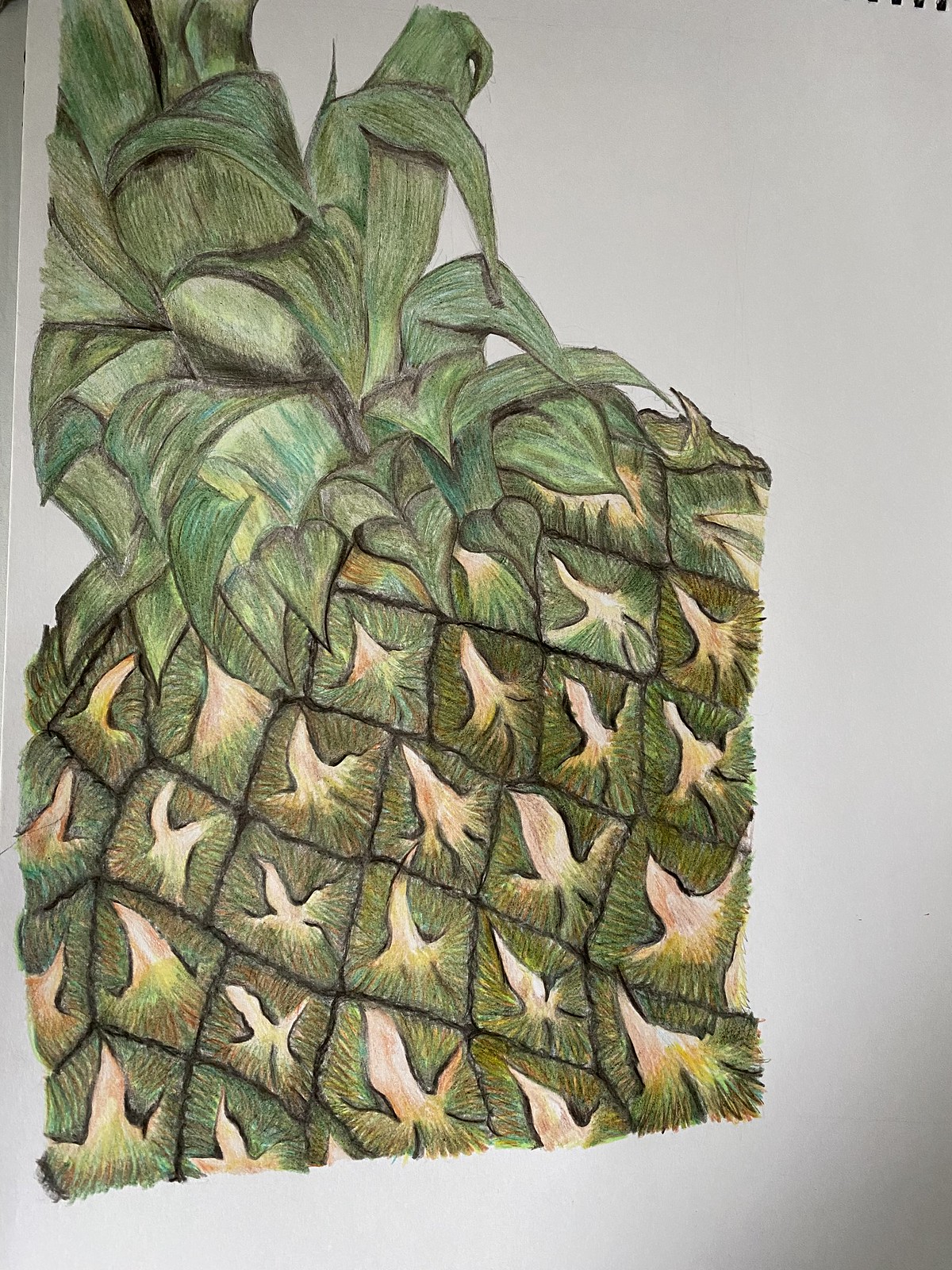This sketch, rendered on white paper, showcases a detailed segment of a pineapple. The artist has focused on a chunk of the pineapple, meticulously illustrating the texture with skilled precision. Using colored pencils, the segment is brought to life with golden and white hues, delineating the diamond-shaped patterns characteristic of the fruit. The crown of the pineapple, often referred to as the "head," is also featured. Its green fronds are shaded intricately with a mix of green, yellow, and hints of black, creating a lifelike appearance. The piece captures the essence of the pineapple's texture and color, providing a vivid depiction of a partial, yet recognizable, pineapple.